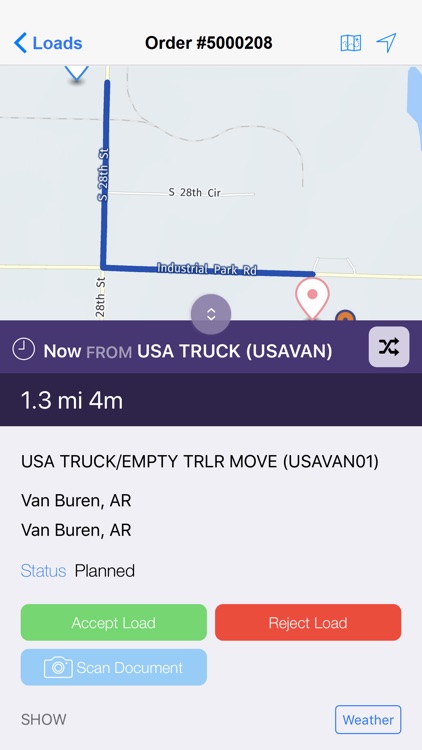The image is a screenshot from a mobile app, likely tailored for trucking logistics, given the information presented in a compact view suitable for a phone or tablet. 

At the top, the header displays text indicating an order number, specifically "Order Number 5,208." To the left of this text is a blue button labeled "Loads," accompanied by a map icon and an arrow.

Beneath the header, the main section features a map showcasing a highlighted route marked by a blue line in the shape of an "L." Key street names such as "Industrial Park Road" and "South 28th Street" are visible on the map.

Below the map, there is detailed trip information. It states the origin and destination, "USA Truck, USA Van," along with distance and estimated travel time: "1.3 miles, four minutes." Additional details include the load status, truck type (USA Truck-Empty, TRLR Move, USA Van 01), and location in Van Buren, AR, with the status marked as "Planned."

At the bottom, there are three prominent buttons for user interaction: 
- A green "Accept Load" button
- A red "Reject Load" button
- A blue "Scan Document" button

Additional options include buttons labeled "Show" and "Weather," offering more features likely pertinent to load details and current weather conditions.

Overall, this image illustrates a trucking application interface, providing users with essential information for managing and selecting truckloads, including route details, load specifics, and interactive options for load acceptance and documentation.